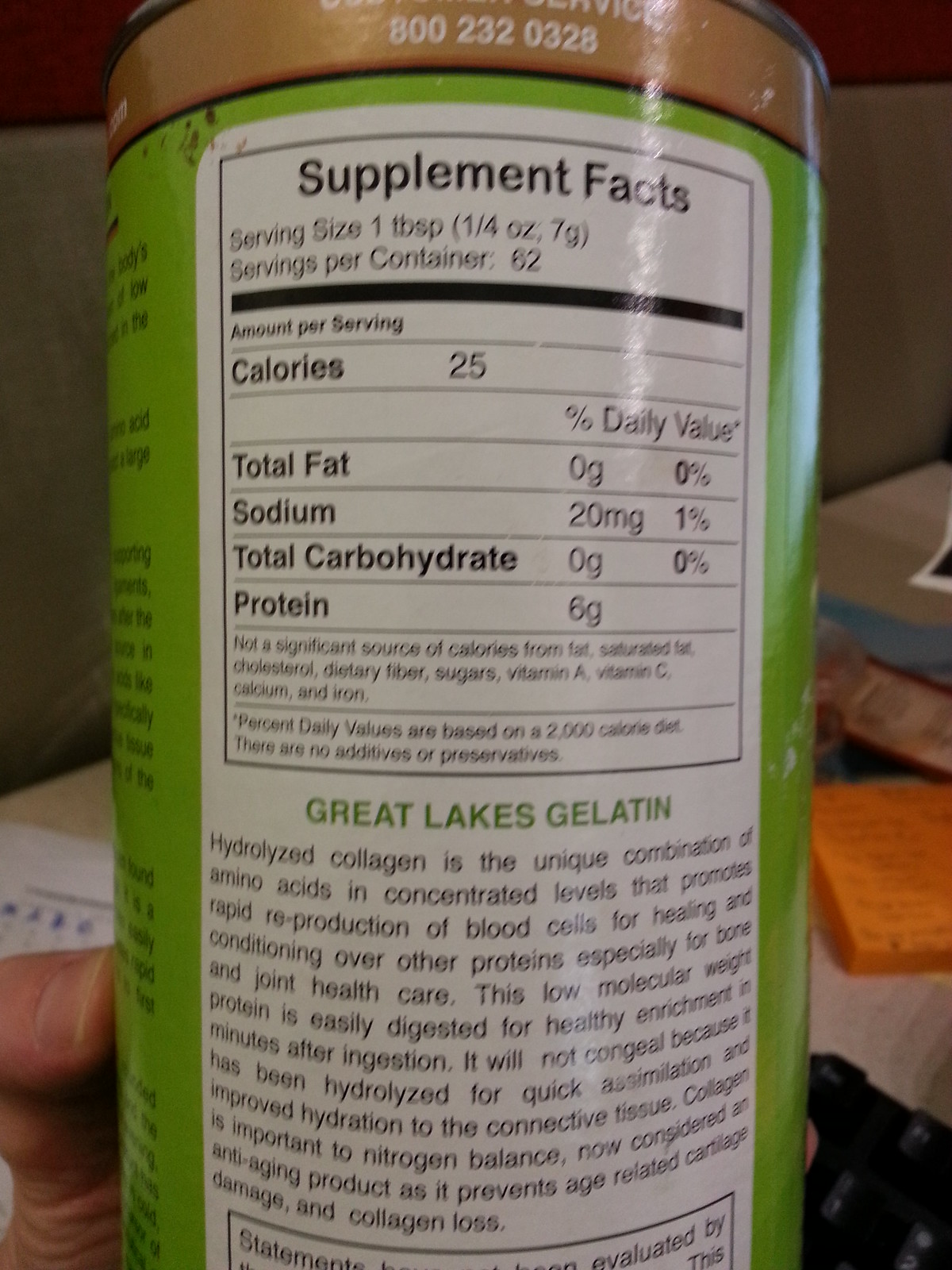A plastic canister labeled "Great Lakes Gelatin" is prominently featured in the foreground, being held by a hand. The cylindrical container, which has a green label, is turned to display nutritional information, showing that each serving contains 25 calories and zero grams of total fat. The central part of the label clearly states "Great Lakes Gelatin," along with other product details. In the background, a countertop cluttered with various items—an orange square, several packages, and a notebook—can be seen. The corner of a black object is also visible in the right-hand side of the image, contributing to the overall context of an everyday kitchen scene.